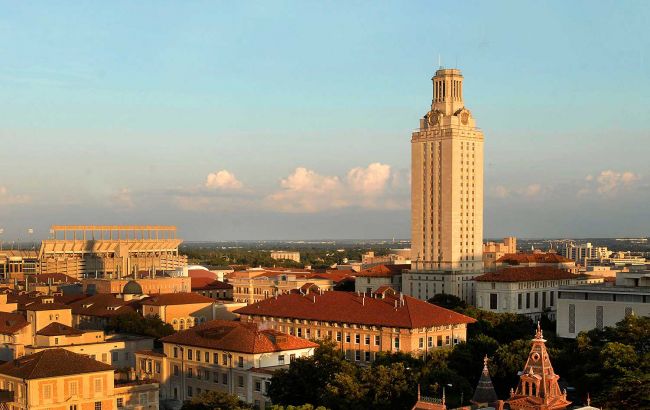In this outdoor color photograph taken on a clear sunny day, we are presented with a detailed and vibrant view of a town from a high vantage point. Dominating the scene towards the center-right is an imposing, rectangular stone skyscraper that soars approximately 20 to 25 stories into the sky. This tall, tan-beige building features a distinctive clock tower at its peak, making it stand out markedly from the surrounding structures. 

In the foreground, several four to five-story buildings with reddish-brown roofs exhibit a harmonious blend of yellow, white, and beige hues. These shorter buildings create a layered contrast against the prominent skyscraper. To the left of the scene, a stadium is noticeable, with its structure extending towards the background. The far distance reveals a flat horizon lined with some greenery and grass. 

The sky above is mostly blue, adorned with low-lying, cotton-like white clouds. In the bottom-right corner of the image, there's a modern building with a triangular top, adding a touch of architectural diversity to the cityscape. The overall lighting suggests a golden hour ambiance, with a warm hue casting pronounced shadows and giving the entire scene a slightly golden glow. This photograph captures the essence of a tranquil, sunny day in this quaint yet dynamic town.